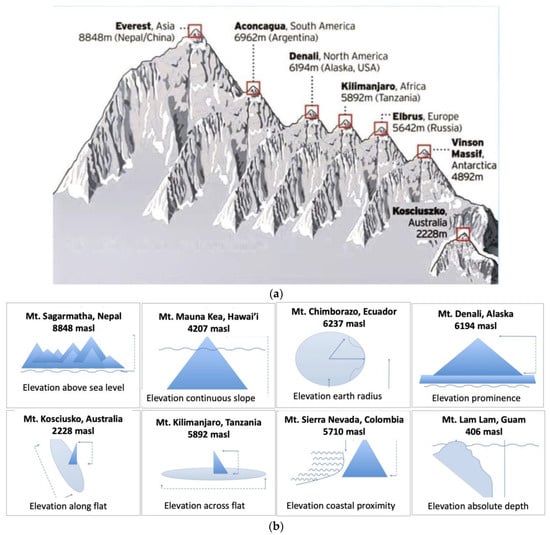This image, seemingly a snippet from a geography book, features a detailed infographic comparing the heights and characteristics of the world's tallest mountains. In the top half (labeled 'A'), it showcases an illustration with seven major peaks: Everest, Aconcagua, Denali, Kilimanjaro, Elbrus, Vinson Massif, and Kosciuszko. Each mountain is encased in a red square, with annotations providing their heights and geographical locations. 

Beneath this (labeled 'B'), the infographic presents a grid with eight rows and two columns, each cell containing additional detailed illustrations in varying shades of blue. These illustrations convey various aspects of elevation for different mountains. For example, it highlights the continuous slope of Mauna Kea in Hawaii and the earth's radius elevation for Chimborazo in Ecuador. Other notable mentions include the elevation prominence of Denali in Alaska, coastal proximity of Sierra Nevada in Colombia, and absolute depth elevation of Mount Lam Lam in Guam. Each illustration is accompanied by black lettering for easy reference.